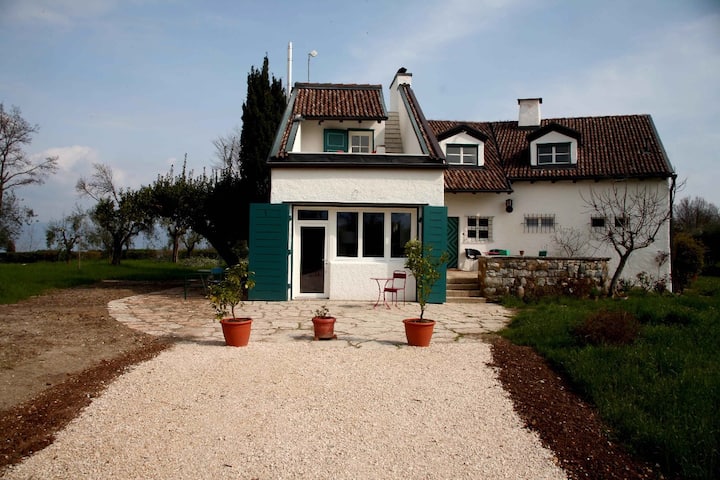This photograph captures a charming, small white cottage with a distinctly Cape Cod architectural style, set under a vibrant blue sky scattered with light, wispy white clouds. The exterior features dark green shutters and a mix of windows, including three on the ground floor alongside a glass front door and another green door. Two dormer windows are visible on the upper level. Leading up to the house is a stone pathway bordered by verdant green grass and some trees. In front of the house, three large terracotta pots with thriving plants add a touch of greenery. A stone patio area with a small table and a single chair sits invitingly to the right of the front door, perfect for enjoying the serene surroundings. To the right-hand side of the driveway, there is a patch of dirt or mud area devoid of grass or stones. The overall scene is picturesque and tranquil, exemplifying a quaint, cozy residence.